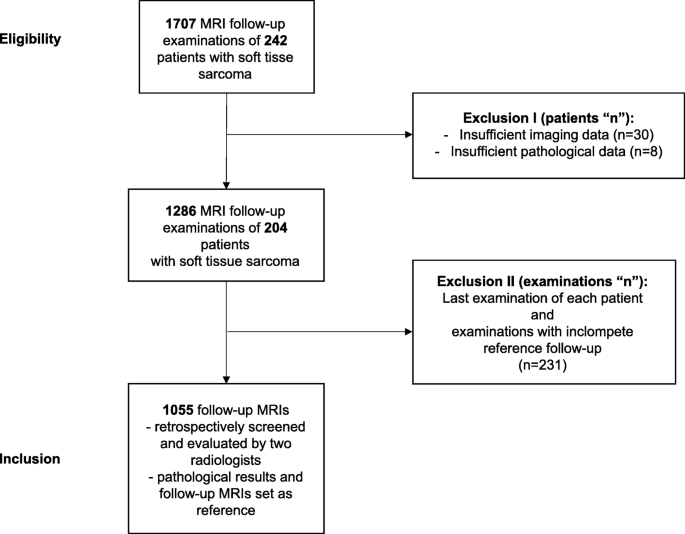The image is a detailed black-and-white flowchart related to MRI follow-up examinations for patients with soft tissue sarcoma, formatted as follows: 

At the top left corner, in black letters, it says "Eligibility," and at the bottom left corner, it says "Inclusion." To the right of "Eligibility," there is a black rectangular box stating "1707 MRI follow-up examinations of 242 patients with soft tissue sarcoma." An arrow from this box points down to a second black rectangle that reads "1286 MRI follow-up examinations of 204 patients with soft tissue sarcoma." 

In the middle of the downward arrow connecting these two boxes, there is a rightward arrow leading to a longer black rectangle labeled "Exclusion 1: insufficient imaging data, insufficient pathological data." 

Below the second rectangular box, another arrow points downwards to a black square with text stating "1055 follow-up MRIs retrospectively screened and evaluated by two radiologists, pathological results and follow-up MRIs set as reference." Between this downward arrow, there is another rightward arrow leading to a black rectangle labeled "Exclusion 2: last examination of each patient and examinations with incomplete reference follow-up." 

This diagram systematically segregates the data into eligibility and exclusion criteria, providing a clear pathway for understanding the process of MRI follow-up examination evaluation.